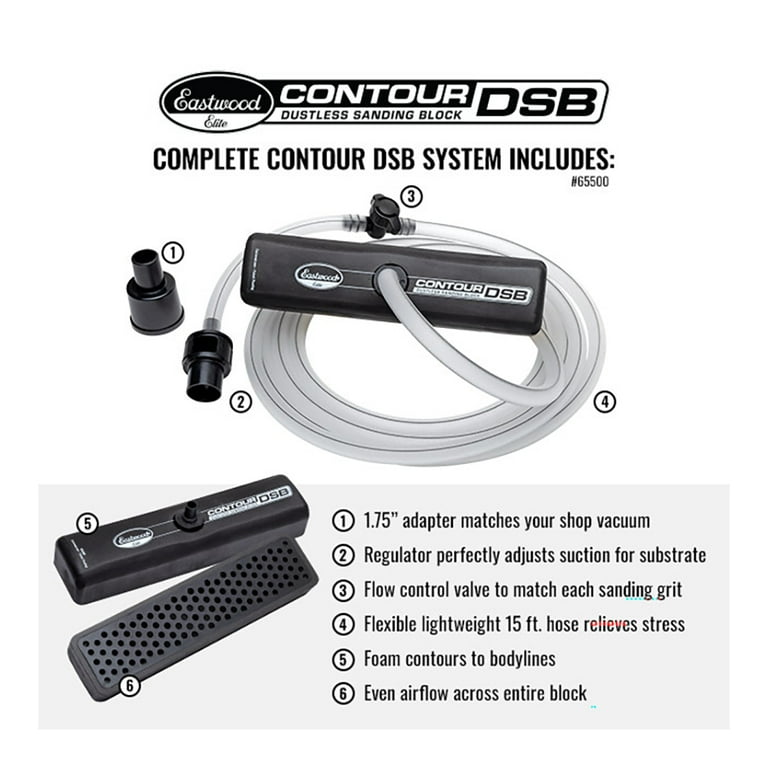This black-and-white advertisement showcases the Eastwood Elite Contour DSB Dustless Sanding Block, meticulously designed for use in auto repair shops. The rectangular sanding block connects to a clear hose equipped with a plug at the end, ensuring a dust-free working environment. Alongside the image, the ad details seven key features: a 1.75-inch adapter compatible with shop vacuums, an adjustable regulator for substrate suction, a flow control valve tailored to different sanding grits, a 15-foot flexible and lightweight hose to alleviate user stress, foam contours that adapt to body lines, and an even airflow across the entire block. Numbered annotations clearly correspond to these features, with visual cues such as the perforated foam block and the top-attached hose, emphasizing the product's comprehensive design and functionality for professional sanding tasks.